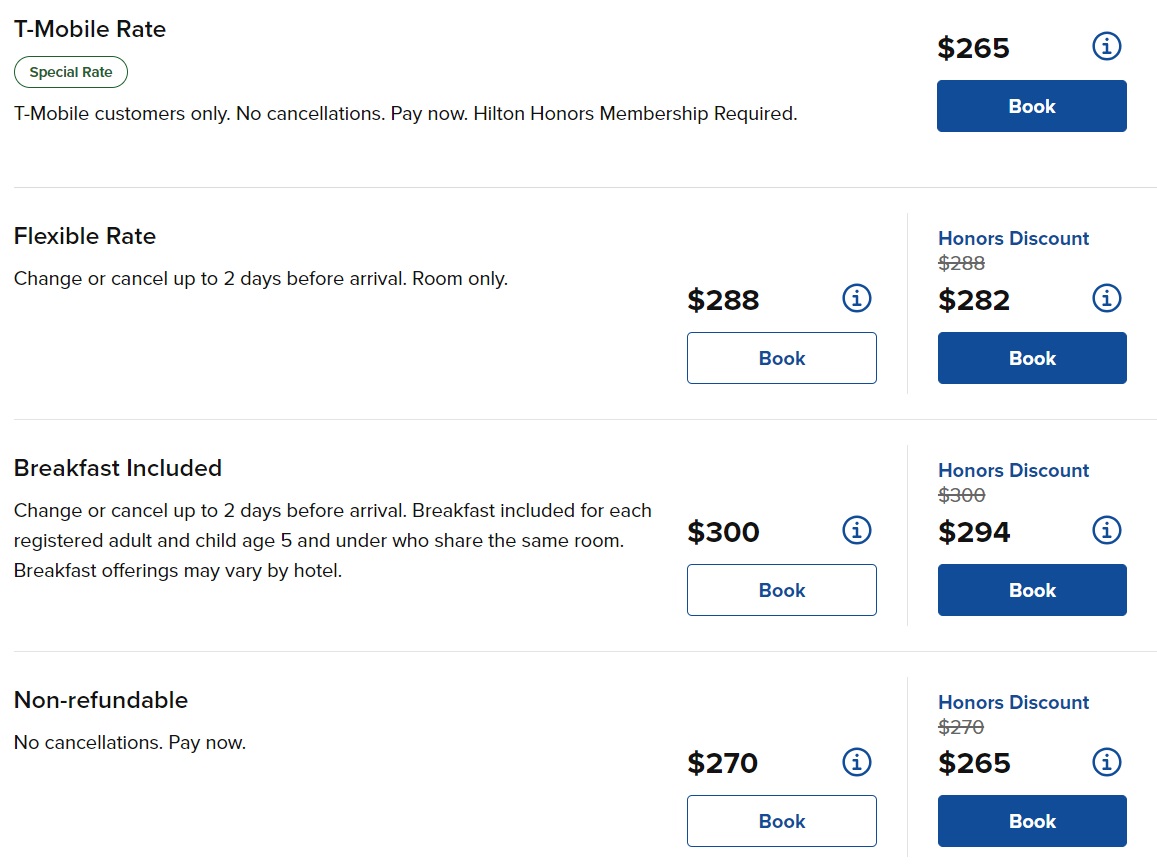This image showcases a screenshot detailing different room rates, prominently highlighting various booking options. At the top, "T-Mobile Rate" is displayed. Below, four distinct rates are presented:

1. **Special Rate for T-Mobile Customers**: 
   - Identified by a green oval shape with "Special Rate" inside it.
   - Exclusive to T-Mobile customers, it requires immediate payment and has no cancellation options.
   - A Hilton Honors membership is necessary.
   - Price: $265.
   - To the right, a blue rectangular "Book" button is featured with an informative "i" icon above it.

2. **Flexible Rate**:
   - Allows changes or cancellations up to two days before arrival.
   - Room-only rate priced at $288.
   - Next to it, an "Honors Discount" is listed at $282, both accompanied by the blue "Book" button.

3. **Breakfast Included**:
   - This rate includes breakfast for $300.
   - With the "Honors Discount," the price is reduced to $294.
   - Both rates have the blue "Book" button associated with them.

4. **Non-Refundable Rate**:
   - No cancellations are permitted and payment is required upfront.
   - The initial price is $270.
   - With the "Honors Discount," this rate is slightly reduced to $265.
   - Both prices are paired with the blue "Book" button.

All options ensure easy booking with highlighted "Book" buttons for user convenience.